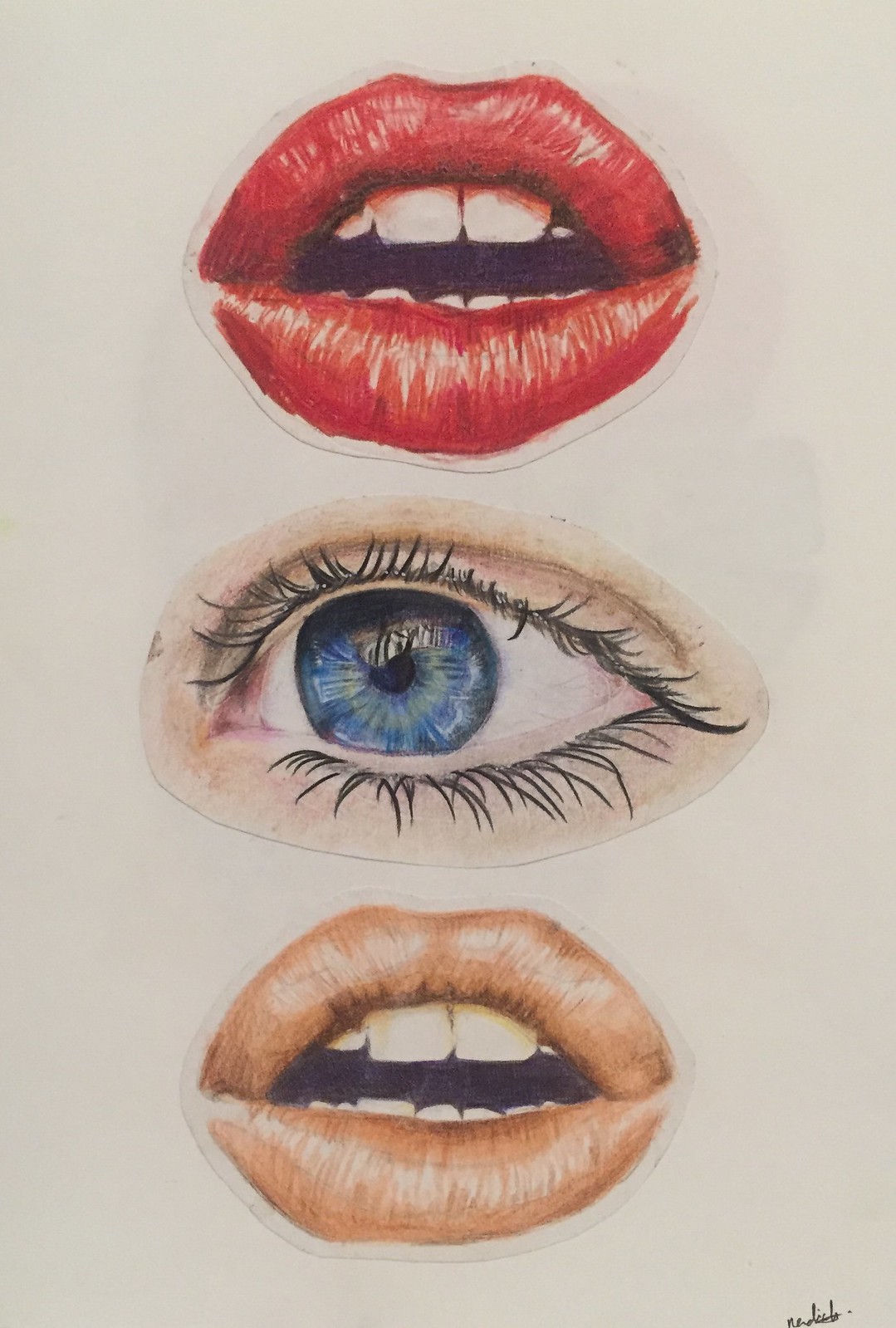The poster features a meticulously arranged graphic image showcasing three distinct human facial elements, each set against an off-white background. At the top center, striking red lips are depicted, painted with vivid red lipstick and revealing a glimpse of the teeth. Positioned in the middle is half of a human eye, primarily the right side, characterized by its vivid blue iris and framed by a dark black eyebrow, indicating a Caucasian individual. Beneath this, the poster displays another close-up of lips in a lighter shade of red or bronze lipstick, with the mouth slightly open to expose the teeth. A small, handwritten signature is present on the right side of the image, although it remains indecipherable due to its size. The entire composition exudes an artistic flair, suggesting it may be a piece from a graphic artist.